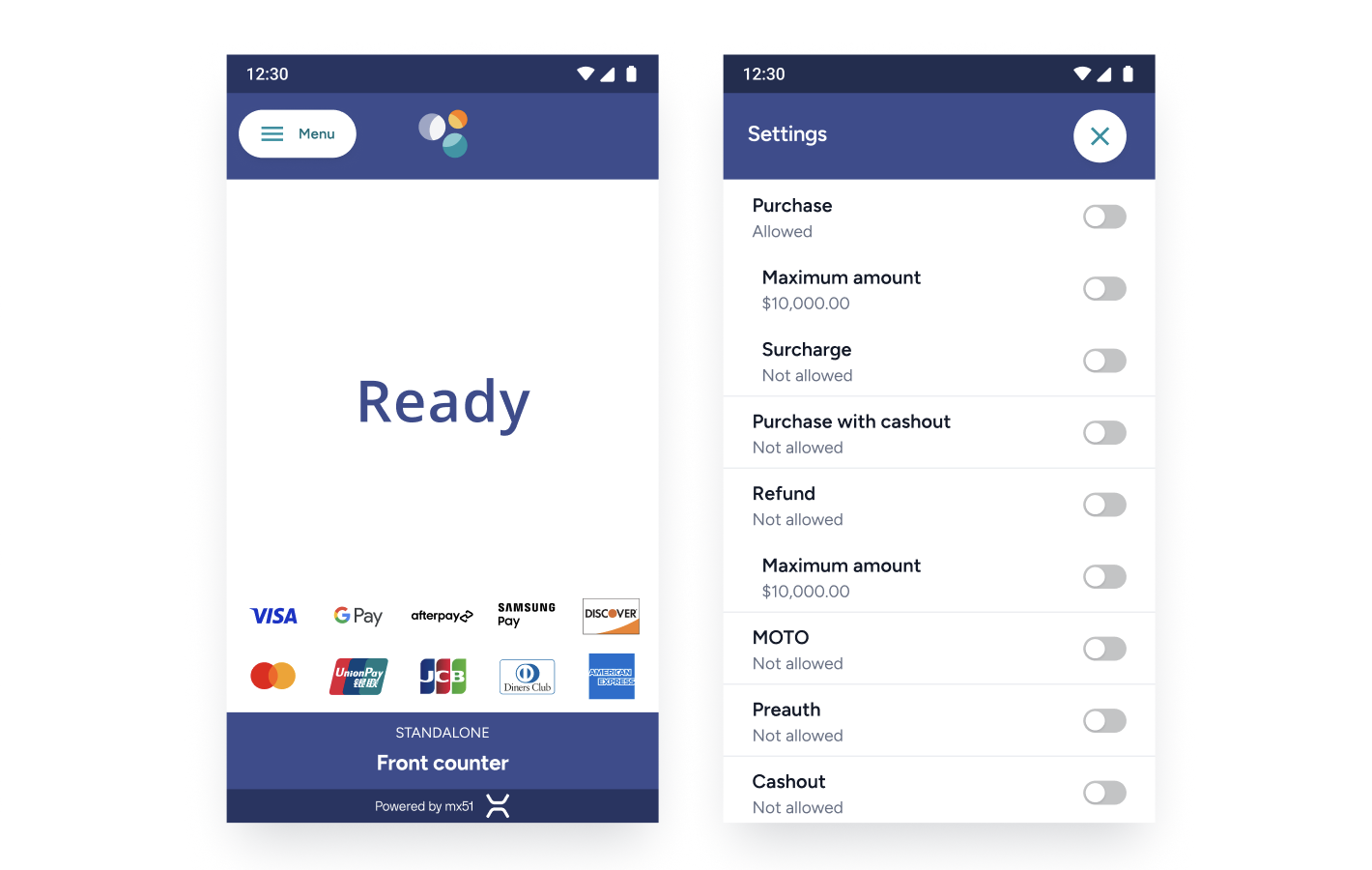This image captures two distinct screenshots with a noticeable gap between them. The screenshot on the left prominently features the word "READY" in large blue letters at its center. Below "READY," various payment options are displayed in two rows, each containing five options. The first row includes Visa, Google Pay, Afterpay, Samsung Pay, and Discover. The second row showcases American Express, JCB, Diners Club, a repeat of American Express, and another unspecified payment card. Beneath these options, a blue banner with the word "STANDALONE" written in the center is visible, followed by a label reading "FRONT COUNTER." At the very bottom, centered, it states "POWERED BY" accompanied by a small logo.

The screenshot on the right is titled "SETTINGS" at the top and features the same blue banner at its header. An X button is located in the top right corner for closing the settings panel. Below the header, there is a vertical list of different settings options, each accompanied by a toggle switch on the right side that allows the user to turn the settings on or off.